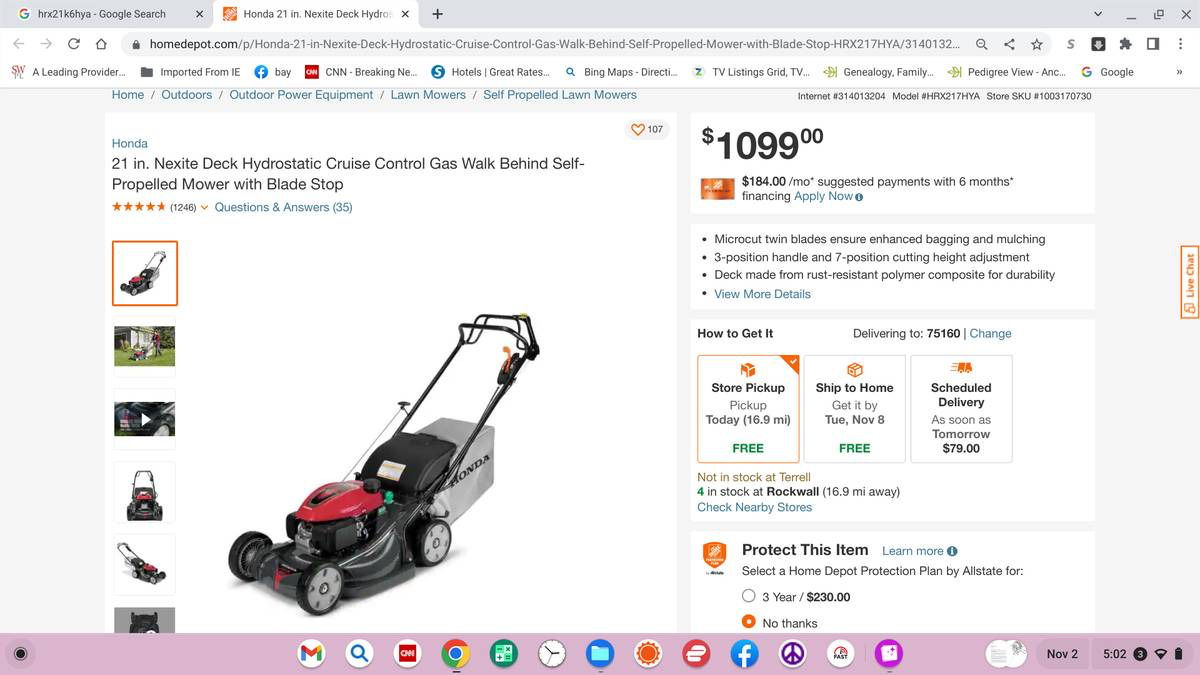This image depicts an online listing for a high-end lawnmower. The product is identified as the "221 NexTile Deck Hydrostatic Cruise Control Gas Walk-Behind Self-Propelled Mower with Blade Stop." The lawnmower itself features a sleek design with a predominantly black body, accented by a touch of red at the top. The chute, responsible for discharging grass clippings, is silver. Displayed prominently in the listing, the price of this advanced mower is $1,999. Below the image, additional product details are available. At the bottom of the screen, a purple bar showcases various app icons, including Gmail, Chrome, and Clark, among others.